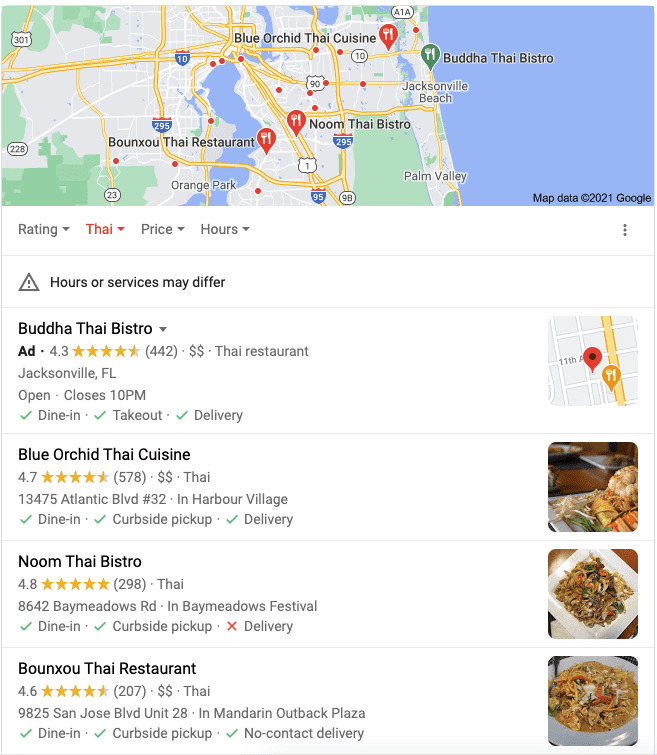The image is a Google Maps search result for Thai restaurants in a coastal area, possibly Florida, indicated by the presence of Jacksonville Beach, Palm Valley, and Orange Park. The top 20% of the image is dominated by an illustrated map showing water bodies to the right, symbolizing the coast, and is marked with various icons and symbols. Notable icons include a green marker for Buddha Thai Bistro, and red markers for Blue Orchid Thai Cuisine, Noom Thai Bistro, and Bun Zao Thai Restaurant, each adorned with a white fork and knife symbol.

Below the map, a sub-menu provides filter options for rating, cuisine type, price range, and business hours, while a three-dot menu lies to the far right. The word "Thai" appears highlighted in red, indicating the selected cuisine.

A thin gray line separates this menu from a caution icon warning that hours or services may differ, followed by another thin gray line.

In the detailed list of restaurants, the first entry is "Buddha Thai Bistro," marked as an ad. It boasts a 4.3-star rating out of 5 from 442 reviews, symbolized by partially filled stars. The information reveals it is a Thai restaurant located in Jacksonville, Florida, with operating hours until 10 p.m., offering dine-in, takeout, and delivery services. To its right is a Google Maps thumbnail with a red marker.

Following are listings for three other restaurants without ad labels:
1. **Blue Orchid Thai Cuisine**: Rated 4.7 stars, located at 13475 Atlantic Boulevard, #32 in Harbor Village, accompanied by an image of food from within the restaurant.
2. **Noom Thai Bistro**
3. **Bun Zao Thai Restaurant**

Each restaurant entry is neatly separated by thin gray lines, ensuring clarity and ease of navigation.